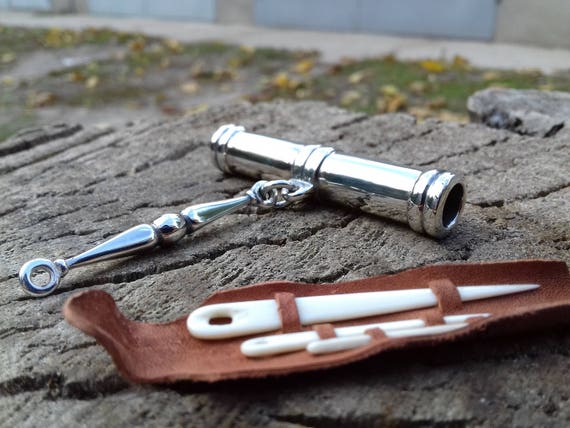The image captures an array of tools arranged on a rough, gravelly ground interspersed with areas of dirt. Dominating the foreground is a russet-colored sheath that holds three white, pointy tools that resemble manicure instruments, neatly affixed in their case. Beside the sheath lies a chrome-colored, cylindrical object that might be a small telescope or a whistle, distinguished by a visible hole on one end and an apparatus perpendicular to it resembling a keychain attachment. A small brown leaf and patches of green grass are visible around the scene, adding a touch of nature to this detailed and somewhat enigmatic arrangement of tools.